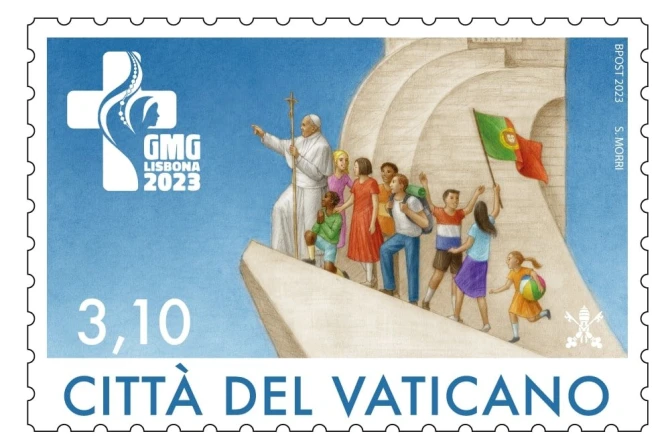The rectangular postal stamp from Vatican City, denomination marked as "3,10 Euros," features a vivid illustration highlighting a significant gathering, likely taking place in Lisbon, as indicated by "GMG Lisbona 2023" in the upper left corner. The focal point is the Pope, dressed in a white robe and holding a cross-topped staff, standing on an inclined rampart. Surrounding him is a diverse group of young adults and children of various ethnicities and hair colors, symbolizing unity and global participation. Key details include a blonde child in a purple dress touching the shoulder of a praying black child in a green shirt and blue shorts. Another female figure in a red dress, a boy in an orange shirt, a youth in a red, white, and blue shirt, and a girl in a light blue shirt and dark blue skirt holding a green and red flag with a central shield, possibly not the Vatican flag, add to the scene. Notably, a little blonde girl in a yellow dress, likely running and holding a beach ball, enhances the lively and inclusive atmosphere. The upper right corner bears the text "B Post 2023 S Mori," likely crediting the artist, S. Mori.